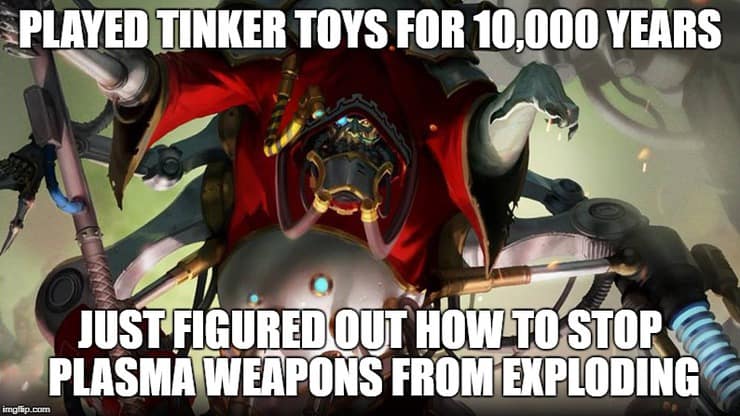In the image, a cartoon depiction of a creature is the central focus. The creature, adorned in a red cloak, has green arms extending forward, with the right arm ending in sharp claws and the left arm connected to a metallic, mechanical structure. The face is covered by a gray mask with gold linings, giving it an enigmatic, formidable appearance. The creature's left arm secures a mechanical extension resembling a shock absorber with illuminated circles at the end. Below this, brown bars and a blue hydraulic line extend downwards. Metal piston legs either support the creature or indicate it is riding a mechanical contraption, which adds to its menacing and robotic image. The backdrop shows indistinguishable contraptions in the upper right. White text overlays the image, reading "Played Tinker Toys for 10,000 years" at the top and "Just figured out how to stop plasma weapons from exploding" at the bottom. In the very bottom left corner, tiny white letters spell out "IMGFLP.com."